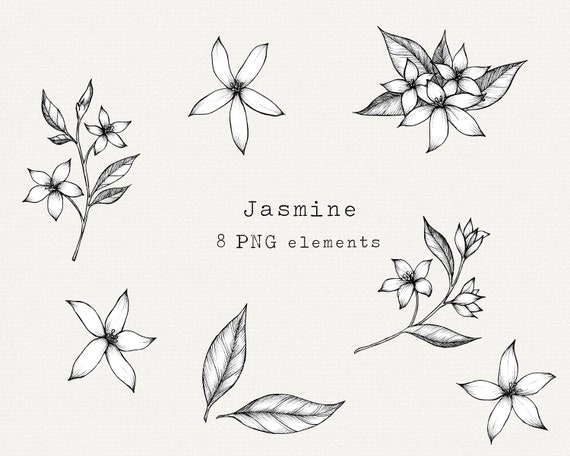The image on a light gray, nearly square background appears to be a delicate advertisement or card showcasing botanical elements. The central focus is on the black text displaying "Jasmine" at the top, followed by "eight PNG elements" underneath. The image is adorned with a series of black and white drawings of flowers and leaves, presumably jasmine. 

In the upper left corner, a curving stem extends leftward, supporting a flower with adjacent leaves, alongside another flower and additional leaves above it. Near the upper center-right, a prominent five-petaled flower is drawn. The top right corner features a detailed black and white illustration of a plant. 

At the bottom left, a flower with five petals is depicted, complemented by two leaves to its right. Above this, another stem with flowers and leaves extends rightward. The bottom right-hand corner exhibits another distinct five-petaled flower. 

The overall arrangement of small white flowers and gray leaves, capturing the subtle and delicate essence of jasmine, overlays the light gray background, enhancing the image's refined and feminine aesthetic.